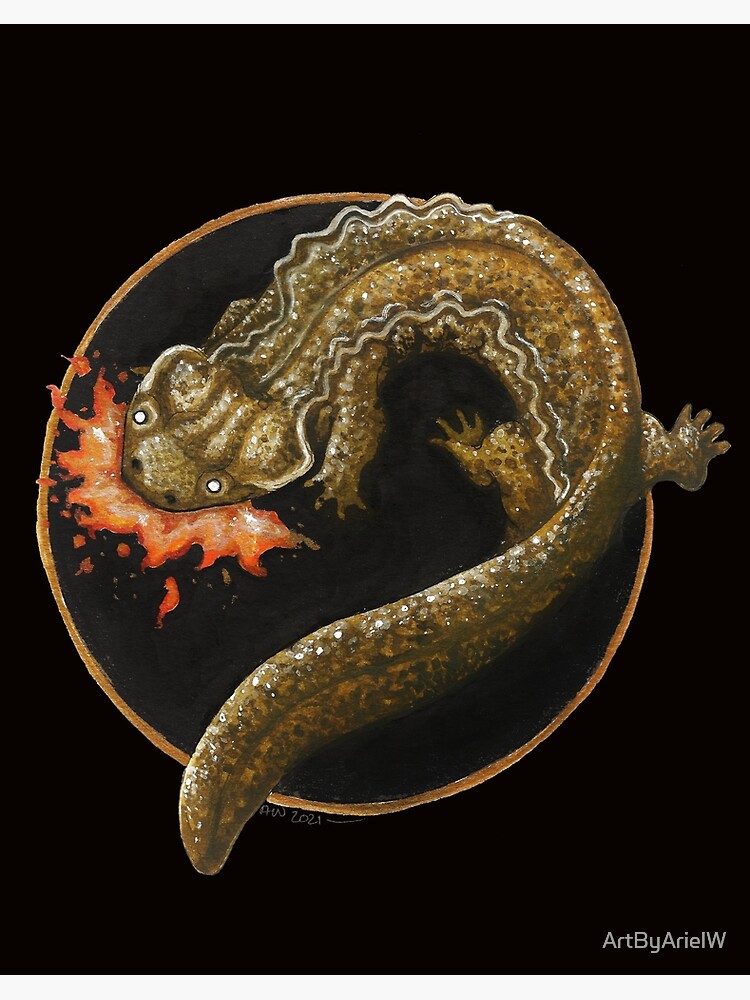The image is a painting signed "Art by Ariel W" in white lettering at the bottom right corner of a black background. Central to the composition is a bronzy gold circle, slightly faded around the edges, containing a creature resembling a small dragon or lizard. The dragon, with a long tail and four legs, is depicted in mottled shades of khaki green and brown. Its body curves to fit within the circle, though one foot and part of the tail extend beyond the boundary. Notably, the dragon has a set of white squiggly lines along its side, a frilly skin flap running halfway down its spine, and two striking white eyes. The head, oriented to the left, is emitting vibrant flames in shades of orange, red, and tangerine, contributing to the dynamic quality of the piece. The image suggests the dragon is breathing fire, creating a sense of movement and energy within the artwork. Additionally, the painting is marked “AW2021” near the bottom, indicating the year of creation.